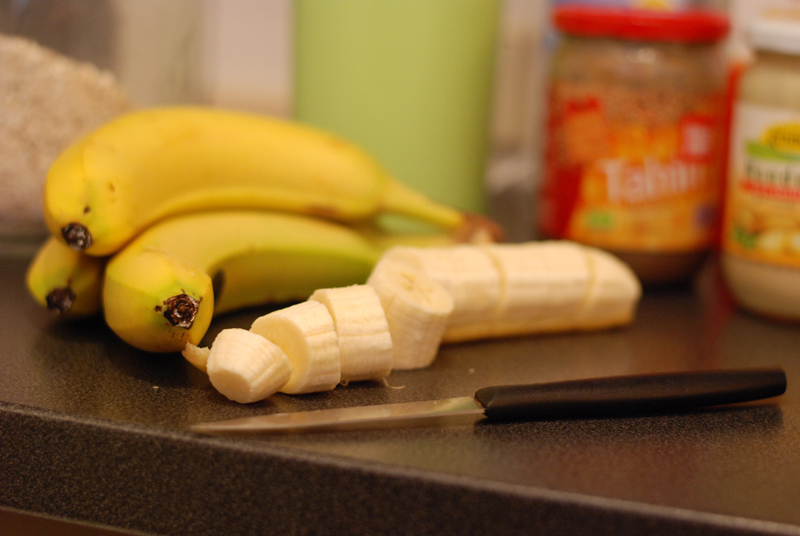In this high-quality image, we observe a kitchen counter featuring a still life arrangement of bananas and other kitchen items. Prominently displayed is a peeled banana, sliced into bite-sized sections, next to a knife with a black handle. Adjacent to the sliced banana, a trio of bananas remain connected, showcasing their vibrant yellow hue. In the blurred background, a container possibly holding rice cereal is visible. Additionally, there is a green cylindrical container whose contents are indiscernible. Towards the upper right section of the image, two jars are present: the one on the left has a red lid with a red and yellow label, partially readable as "TAH," while the jar on the right features a white lid and a green, white, and red logo.